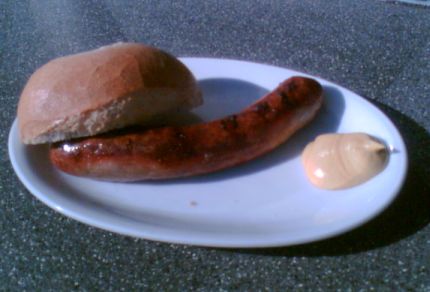This color photograph captures a simple yet appetizing meal set against a speckled gray countertop. The focal point is a plain white dinner plate, which holds three distinct items. At the top left, there's a half roll with a golden-brown crust. Dominating the center is a grilled sausage or hot dog, visible with grill marks that hint at its savory flavor. To the right of the sausage is a dollop of a light mustard-colored condiment, perfect for dipping. The overall composition highlights a minimalist but inviting presentation.